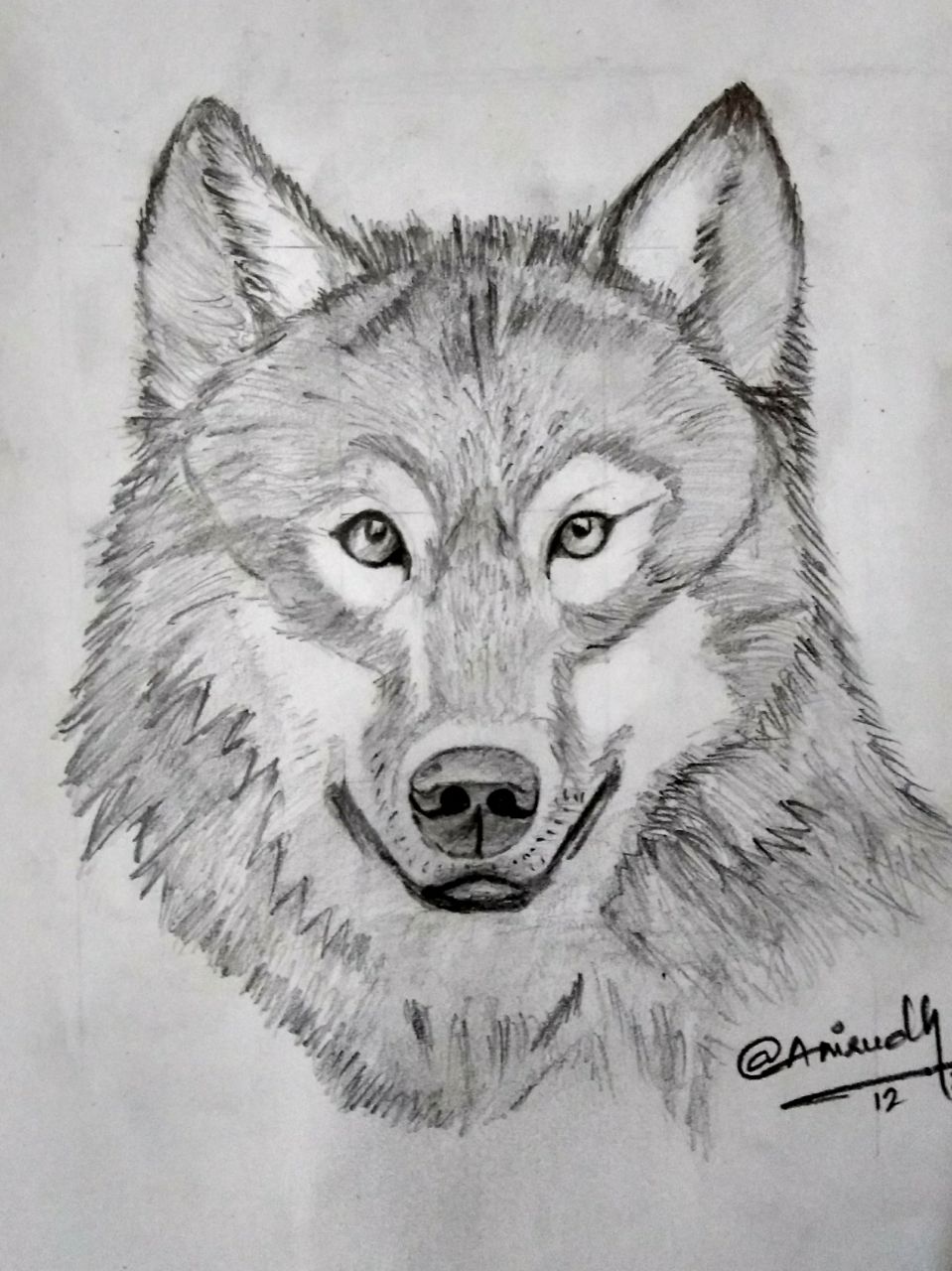This detailed pencil drawing showcases a wolf's head, meticulously rendered with impressive attention to detail. The wolf is depicted facing forward, creating an intense and engaging gaze that seems to capture the viewer. The artist has skillfully drawn the distinctive features of the wolf, including its sharp ears, detailed nose, and expressive mouth. The shading is expertly applied, adding depth and texture to the fur, which enhances the lifelike quality of the piece. In the bottom right-hand corner, the drawing is signed in cursive as "Aamirudy" and is marked with the number 12, indicating either the year of creation or the artist's age. This striking portrayal of a wolf's head is a testament to the artist's talent and technique.